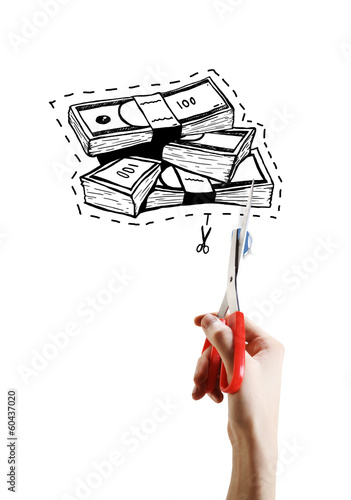The image is a blend of clip art and lifelike photography. The central focus is on four crisscrossed wads of money, each wrapped with bands and displaying the number 100 in black and white cartoon style. These stacks of cash are surrounded by a dotted line border with scissor icons, indicating they are meant to be cut out. The background is a stark white, overlayed with translucent diagonal watermarks that read "Adobe Stock." In the lower section of the image, a realistic human right hand is grasping a pair of open scissors with red handles, poised to cut along the dotted line. The hand and scissors contrast sharply with the cartoonish money above. Additional text reading "Adobe Stock" appears vertically in the very left corner, accompanied by a hashtag and number, creating a detailed and visually engaging stock photo.